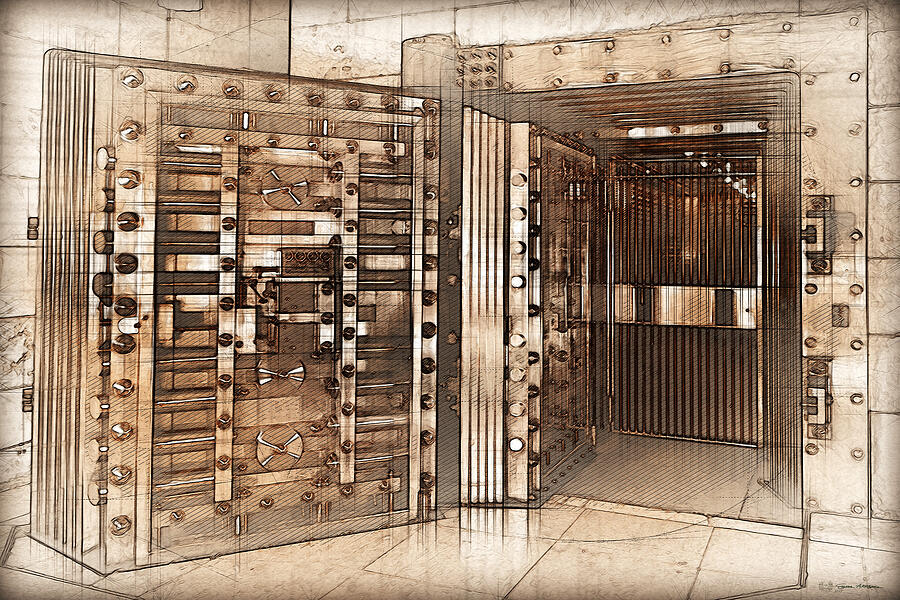This is a highly detailed, sepia-toned illustration of a bank vault door. On the left, a massive, multi-layered metallic door stands ajar, revealing an interior still secured by a cage-like gate, adding an extra layer of security. Both the floor and walls of the vault are composed of rectangular tiles, and the entire image is rendered with stylized, hand-drawn lines in shades of brown and white, lending it a distinctive, copper-colored appearance. The perspective is from outside the vault, emphasizing the formidable, thick, and intricately designed door which underscores the vault's impregnable nature.